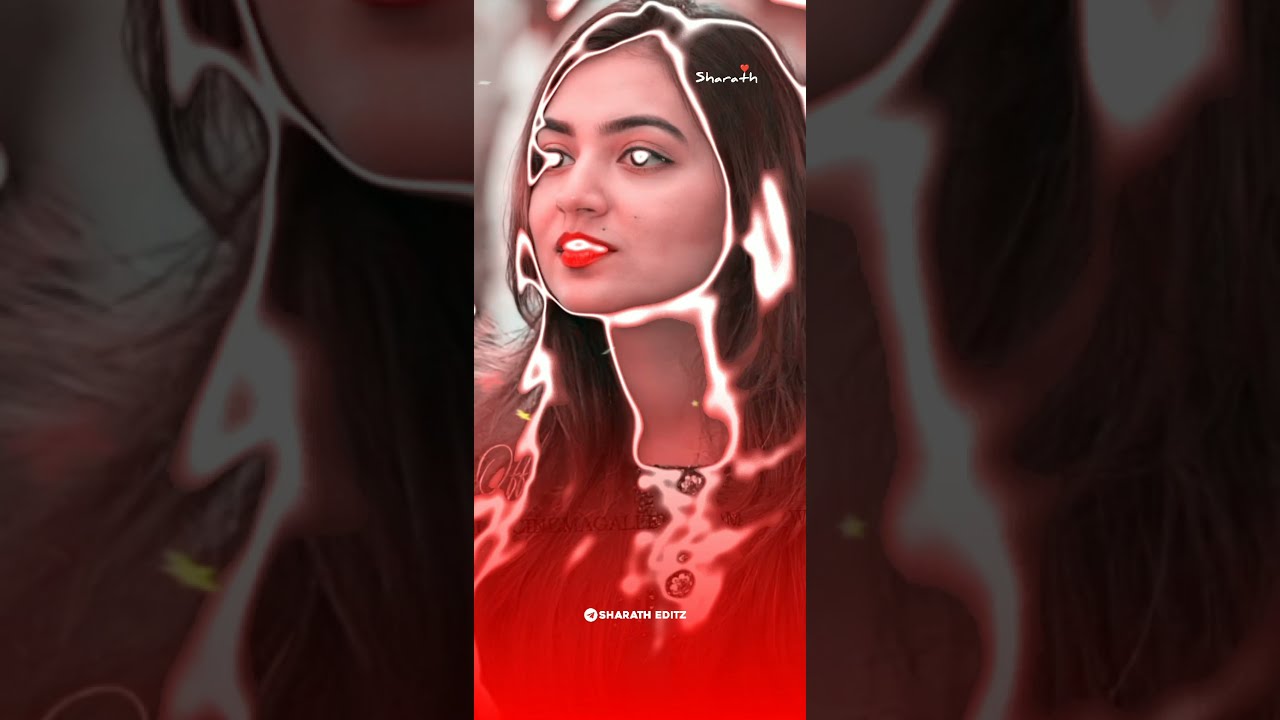This image features a woman prominently positioned in the center, her face serving as the focal point. The entire image has been heavily edited with computer graphics, resulting in a stunning, almost ethereal appearance. Her face, hair, and neck are all surrounded by a glowing white aura, imparting a surreal quality to her features. The woman's eyes and open mouth emit an intense, unnatural white glow, extending even to her teeth. She is wearing striking red lipstick, which stands out against the otherwise monochromatic enhancements. Her brown hair, interwoven with shiny white strands, falls to her shoulders and is parted to the side.

The format of the image suggests it was originally captured in a vertical video mode, possibly from a platform like TikTok, but it's presented here in a horizontal, landscape orientation. This results in a narrow, centralized image of the woman flanked by close-up sections of the same photograph. These side sections mostly capture her hair and part of her illuminated aura, providing a zoomed-in continuation of the central figure. At the bottom of the image, a red element along with the mention of someone's name can be seen, adding a touch of color to the otherwise darkened and digitally enhanced background.